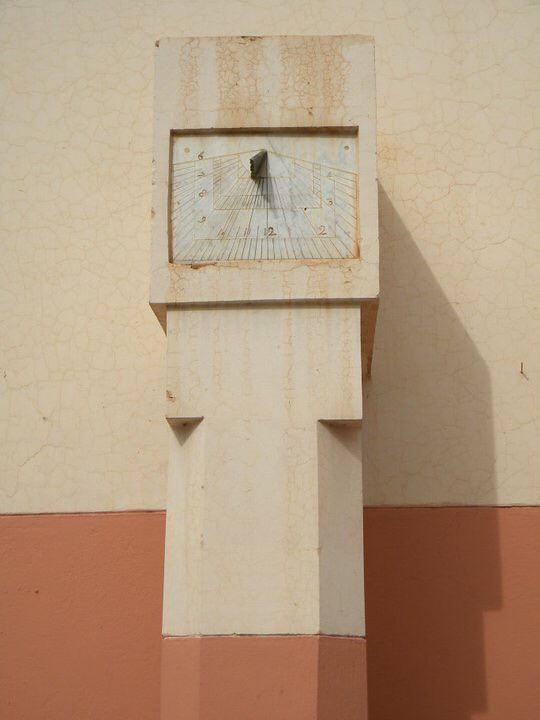This image portrays an ancient sundial mounted on a three-dimensional, rectangular pillar. The sundial, carved with meticulous detail, features numerous lines and small numbers designed to cast and read shadows for timekeeping purposes. The pillar itself is a tannish beige color, providing a stately and weathered look that speaks to its historical significance. The base of the pillar stands on a vivid, reddish-orange platform, which contrasts sharply yet harmoniously with the pillar. The background wall mirrors these colors, with a tan upper portion and a reddish-orange lower portion, enhancing the cohesive aesthetic of the scene. A prominent shadow is cast to the right of the sundial, adding depth and dimension to the image, suggesting the sundial is still functional and engaged with its celestial purpose. This captivating artifact provides a fascinating glimpse into the technological ingenuity of an ancient society.